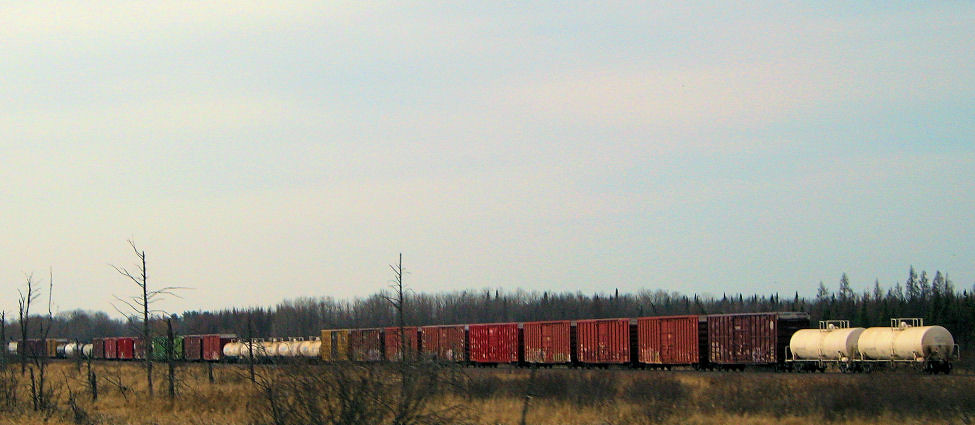In this wide-angle landscape photograph, a cargo train stretches almost the entire width of the image, starting near the bottom right and extending towards the distant background on the left. The train is composed of various dilapidated and weathered cars, predominantly in shades of brick red, green, and cranberry, interspersed with white cylindrical tank cars meant for transporting liquids or gases. The train cars and tankers vary in number, with approximately ten red cargo cars, followed by clusters of tankers and additional mixed cargo cars further along the track.

The foreground showcases a desolate, grassy plain with knee to ankle-high grasses that are primarily dead or dark green in color, suggesting a fall or winter setting. Sparse, leafless trees scatter the area, implying a recent wildfire or harsh seasonal impact. Further back, a line of bare pine trees add another layer of depth to the scene. The sky above dominates the top two-thirds of the image, appearing bright blue but slightly hazy with patches of wispy, grayish-white clouds, contributing to the overall muggy atmosphere. The photograph captures a vivid, somewhat melancholic landscape marked by the stark contrast between the weathered train cars and the surrounding natural environment.